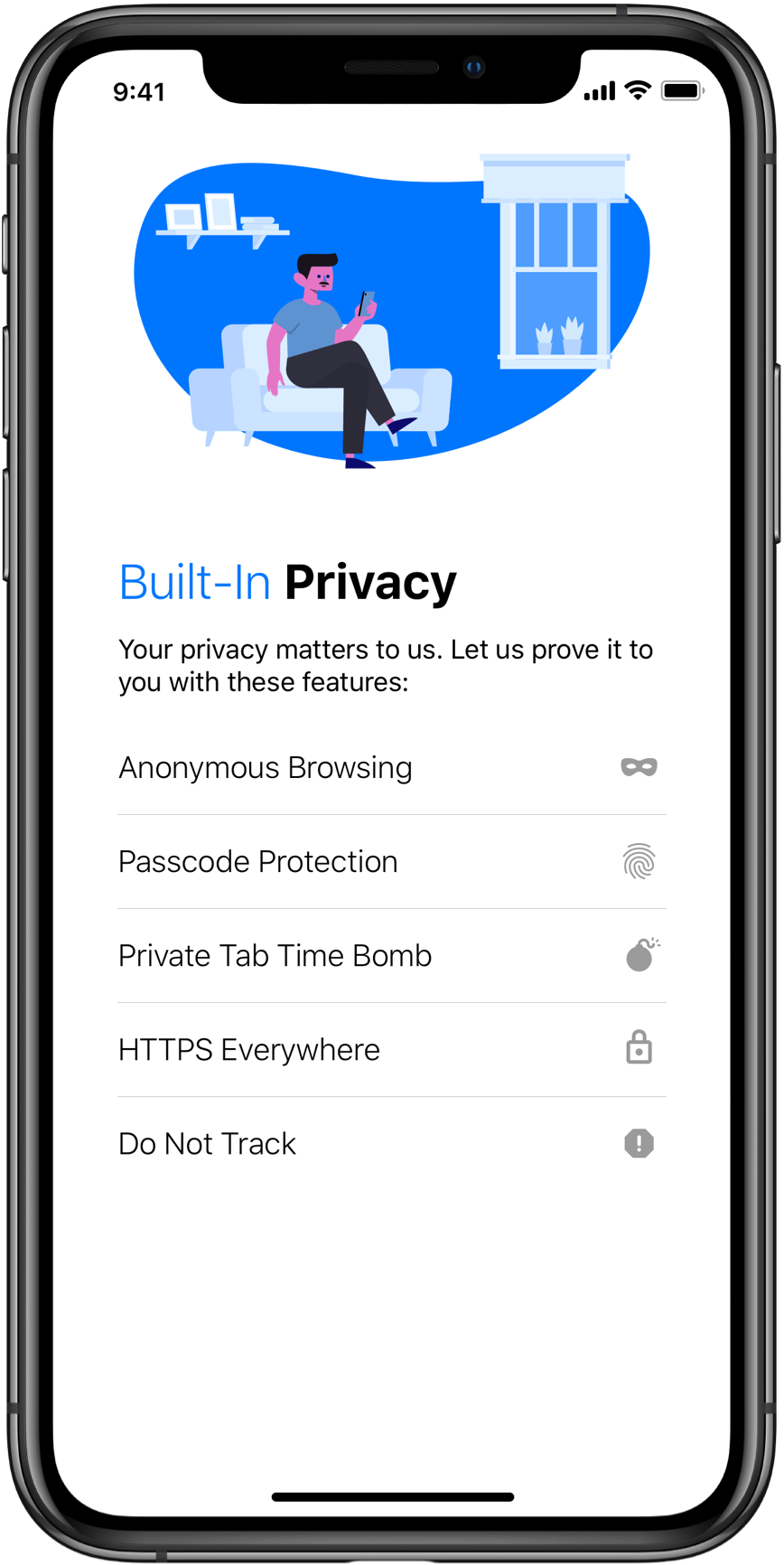This image appears to be a simulated screenshot designed to resemble a cell phone advertisement. The phone has a sleek gray-black border, complete with a notch at the top displaying the time '9:41,' a Wi-Fi symbol, and a battery icon. The screen features a vibrant illustration of a stylized character in a casual blue shirt, black pants, and blue shoes, seated on a white couch while holding a cell phone.

Above the character, a white shelf holds a picture frame and several books. A white window with plants in various shades of white and blue is situated nearby. A prominent blue circle accentuates the upper portion of the image.

Below the illustration, the text reads "Built-in Privacy" in blue and black fonts, followed by a tagline: "Your privacy matters to us. Let us prove it to you with these features." The list of features includes:

- Anonymous Browsing (accompanied by a bandit mask icon)
- Passcode Protection (fingerprint icon)
- Private Tab Time Bomb (bomb icon)
- HTTPS Everywhere (padlock icon)
- Do Not Track (stop sign icon with an exclamation mark)

Additionally, the phone's side view shows the power button and volume controls. The image is of high quality, emphasizing the sleek design and user-friendly features of the phone.